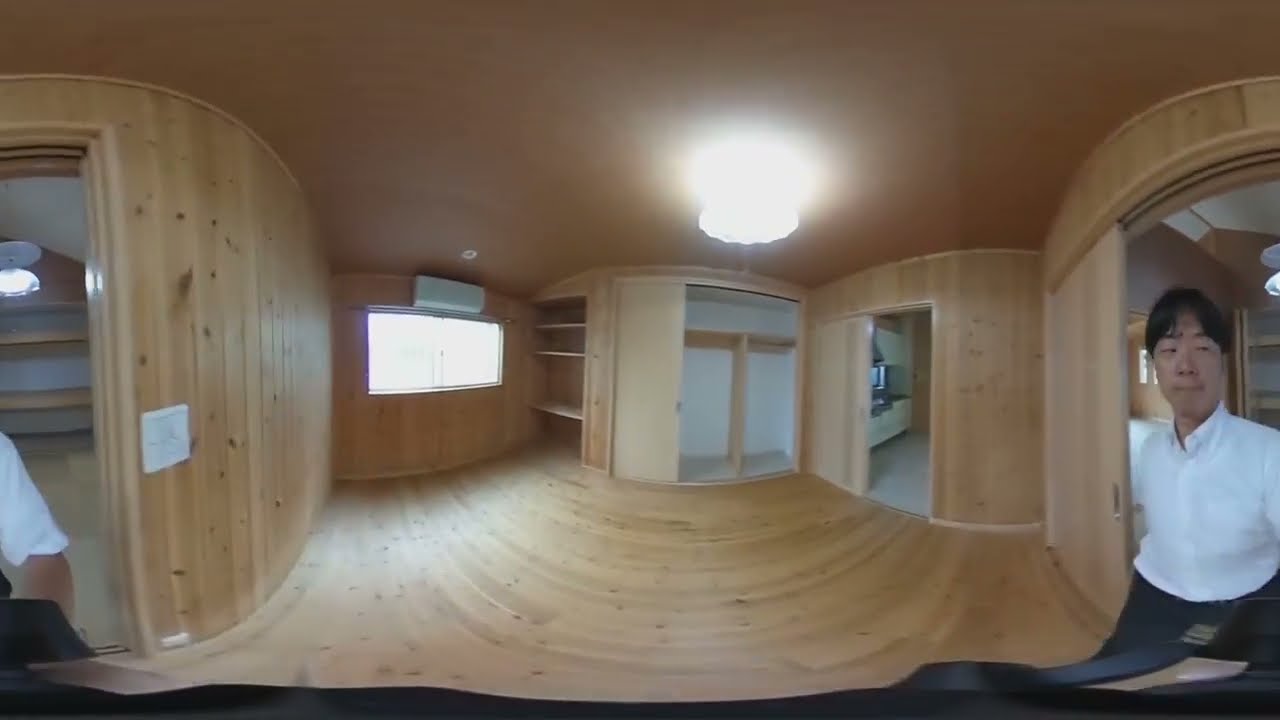This horizontal rectangular image captures an indoor scene bathed in darkness, suggesting it was taken with an unusual lens that accentuates the shadows. The setting is an empty house, possibly an apartment or flat, featuring a mix of beige, light brown, black, tan, and silver tones throughout the space. Central to the image is a dimly lit area with a couple of television screens framed by white paneling, which may function as drawers, adding an element of utility. Flanking the center are hints of a kitchen setup, including stainless steel appliances and white shelving, subtly highlighted with a light greenish-blue hue. To the left, there's a hallway leading to either a window or door and partially shown, a younger man who appears to be of Oriental descent. On the right side, we see parts of an older gentleman standing near shelving and countertops, possibly kitchen shelves. The light wood flooring, though possibly faux, extends across the scene, enhancing the sense of continuity in this vacant home. The ambient lighting indicates it is daytime, and visible doorways hint at more rooms beyond this shared space.